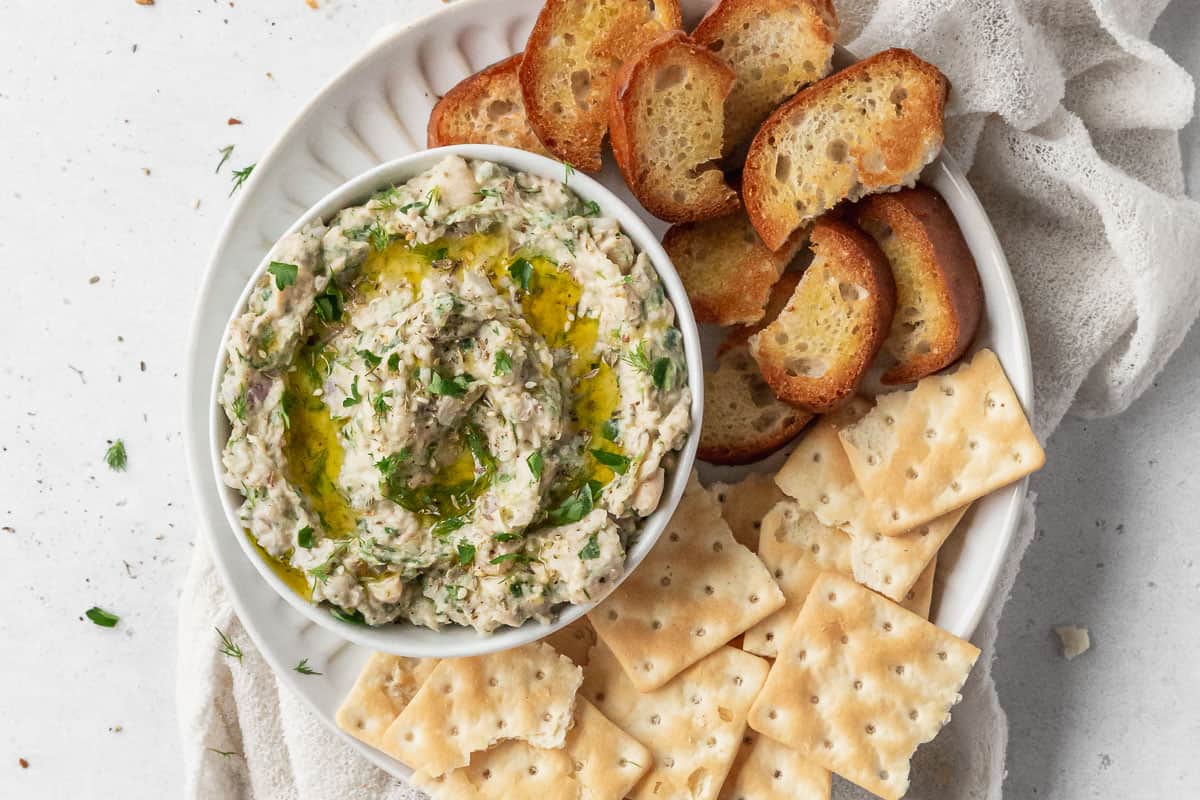The image is a beautifully composed, close-up aerial view of a Mediterranean appetizer platter, arranged with meticulous, yet seemingly effortless detail. A white round plate sits atop a white silk towel draped over a white countertop, creating an elegant, monochromatic backdrop. The plate features two types of crackers: plain graham crackers on the bottom and thick, toasted French bread brioche at the top, both ready to be used for dipping. At the center of the platter is a bowl of dip, possibly hummus or tuna dip, garnished with a drizzle of olive oil and sprinkled with chopped herbs, likely chives or parsley. The surrounding scene is artfully staged, with scattered herbs adding a touch of casual sophistication. The crusty brown of the bread and the vibrant green of the herbs stand out against the predominately white setting, making the presentation both visually appealing and inviting. The image focuses closely on the arrangement, artistically cropping the top and bottom to draw the viewer's eye to the detailed textures and colors of the food.